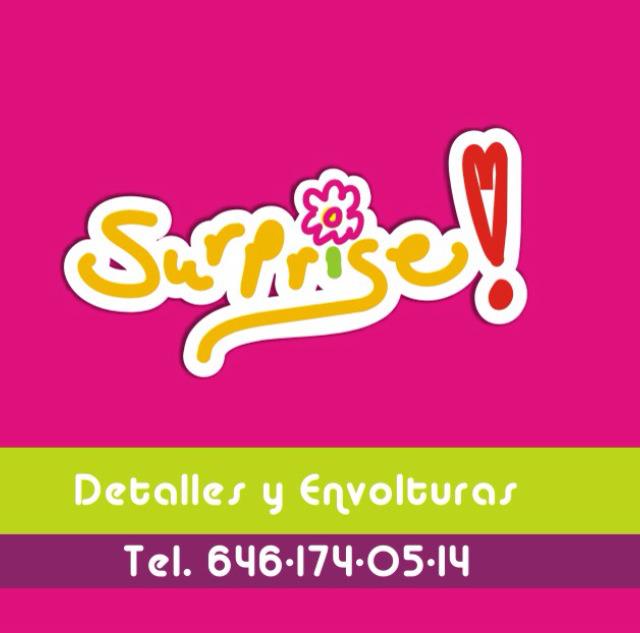This image features a vibrant and eye-catching advertisement set against a bright, hot pink background. Dominating the center is a well-centered logo composed of the word "Surprise" written in gold, accented with a white margin and black outline. The "I" in "Surprise" is uniquely designed; it is green and topped with a pink, hand-drawn flower, creating a whimsical dot. Following the word is an exclamation point, cleverly stylized as a tall, narrow red heart with a dot beneath it, all encased in a white, cloud-like outline.

Beneath the logo, occupying the bottom third of the image, is a horizontal lime green bar with white text in Spanish that reads "Detalles y Envolturus." Below this is a thinner purple bar displaying the telephone number "646-174-0514" in white text, with "TEL." in capital letters preceding the number. The image is a blend of colorful illustration, typography, and graphic design, with additional colors such as orange, yellow, green, lime green, and purple contributing to its lively composition.